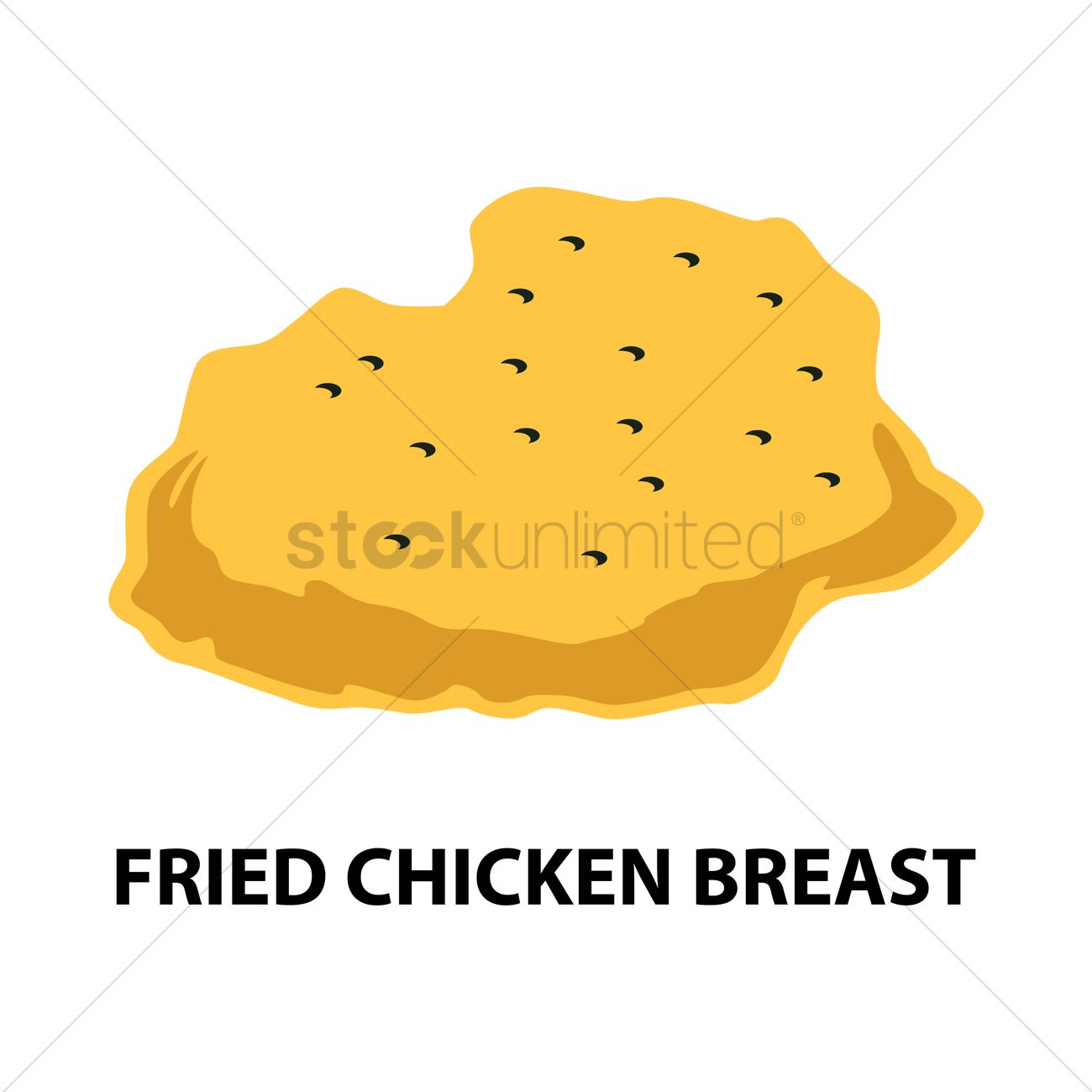The image is an animated clip art labeled "Fried Chicken Breast" with the caption in bold, all-capital, black, sans-serif font underneath it. The background is entirely white. The cartoonish illustration portrays a tan, yellowish, amorphous blob representing a fried chicken breast. The shape is somewhat rounded but irregular and craggy, with shadowed edges. Across the top of the drawing, there are small, black, swoosh-like marks reminiscent of tiny Nike logos. Additionally, the image has a watermark saying "Stock Unlimited," with two diagonal lines forming a cross through the fried chicken breast.